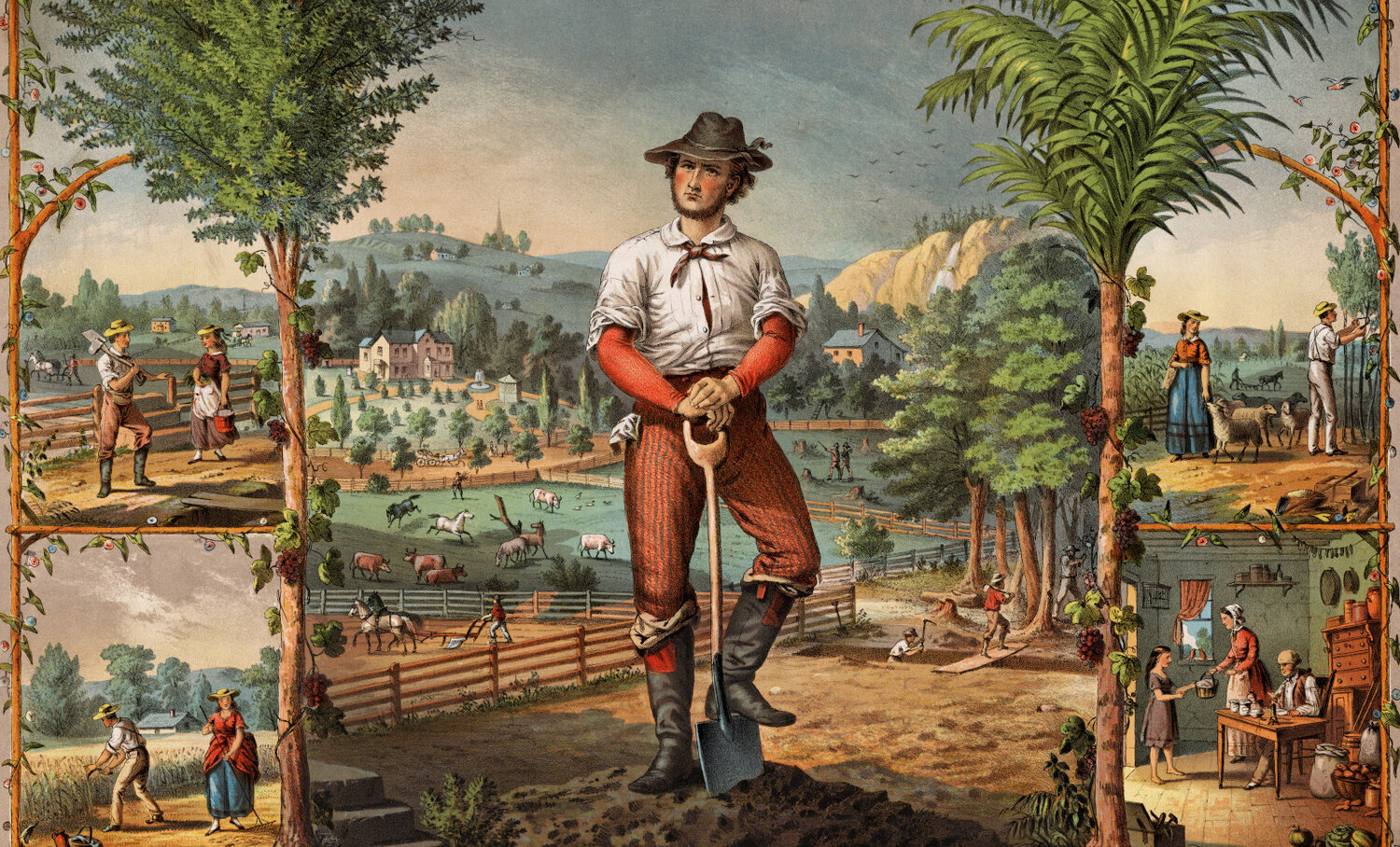This painting, dating back to the early 1800s, portrays a vivid and bustling scene of farm life. At the center stands a young man, dressed in a vividly striped attire: red pants with vertical black stripes, a white overshirt with red sleeves peeking through, black work boots, and a black cap. He grips a shovel firmly, with his left foot pressing down on the blade, ready to dig into the earth. The man's chin is adorned with a beard, adding to his rustic appearance.

The setting around him is a lively farm, characterized by fenced-off areas that contain various livestock, including horses and cows. In the background lies a mansion atop a hill, with smaller houses scattered nearby and tall trees providing a natural backdrop.

Flanking this central image are four smaller vignettes, each capturing different aspects of farm life. In the upper left, a man with a shovel converses with a woman carrying a bucket. Below them, another pair is hard at work: a man harvesting wheat while a woman in a red dress with a blue petticoat rakes up the crop behind him.

On the right side, the upper vignette shows a man tending to a tree while a woman feeds some sheep. Below this, a domestic scene unfolds inside a kitchen: a woman exchanges goods with a young girl while a man sits at a table, seemingly enjoying his lunch. The entire composition is set under an overcast sky, suggesting a gray, somber day, further accentuated by the dark clouds that loom above. The presence of abundant trees and the detailed depiction of both flora and everyday tasks give this painting a rich narrative of early American farm life.